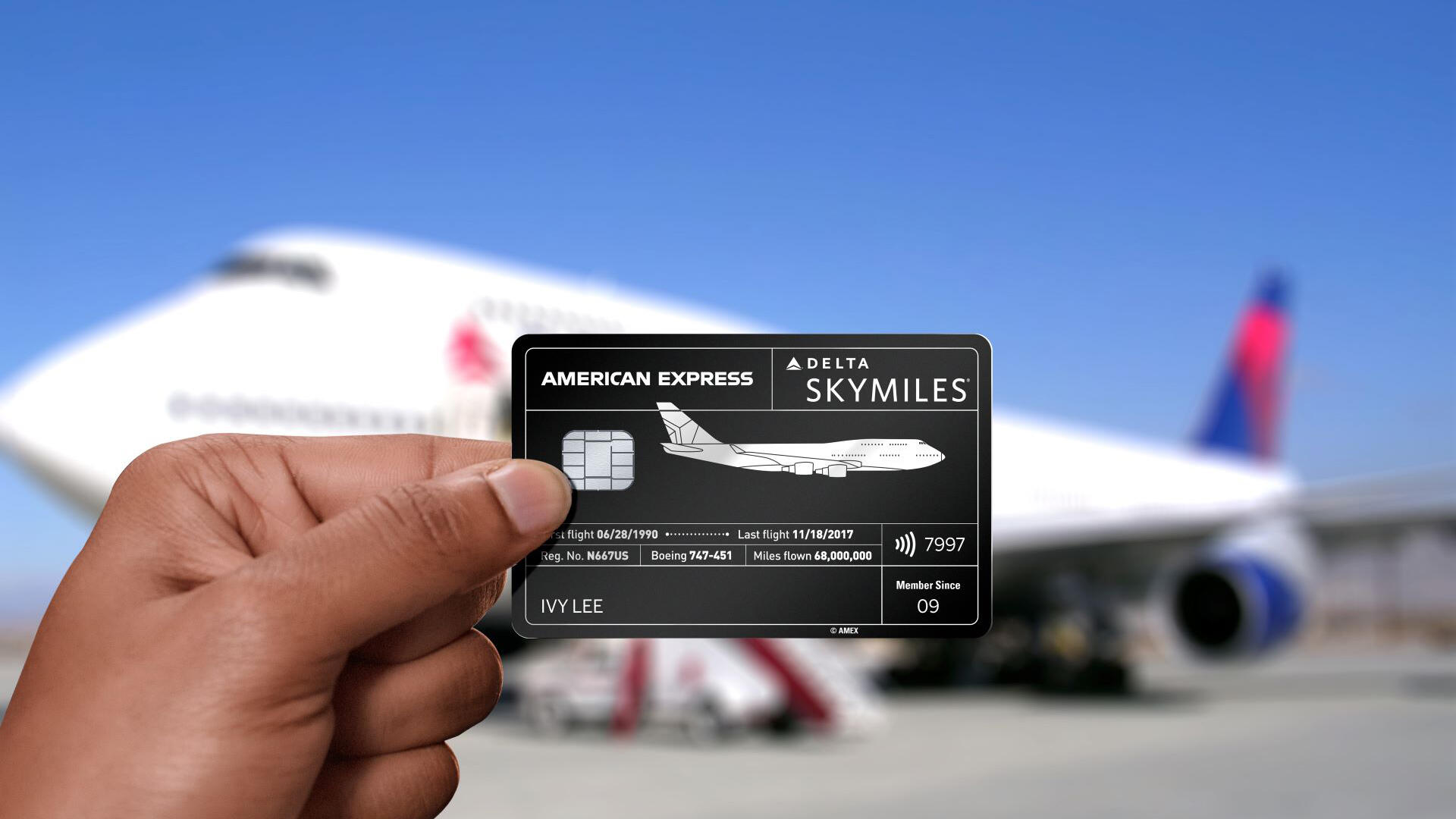The image depicts a detailed close-up of a person’s hand holding a black American Express Delta SkyMiles credit card. In the top left corner, the card is labeled "American Express," and to the right, it reads "Delta SkyMiles" with a small Delta symbol. There is a credit card chip, and next to it, an illustration of an airplane flying to the right. Below, the card details include "First Flight: 06/29/1990" and "Last Flight: 11/18/2017" with an arrow pointing right, and it specifies "Registration Number: N66-7US Boeing 747-451." Further down, it lists "Miles Flown: 68,000,000" and a sound wave icon beside the number "7997." Additionally, it states "Member Since 2009" and the cardholder's name "Ivy Lee." The background is slightly blurred and features a large white, red, and blue airplane facing left, contributing to a bright and naturally lit setting.